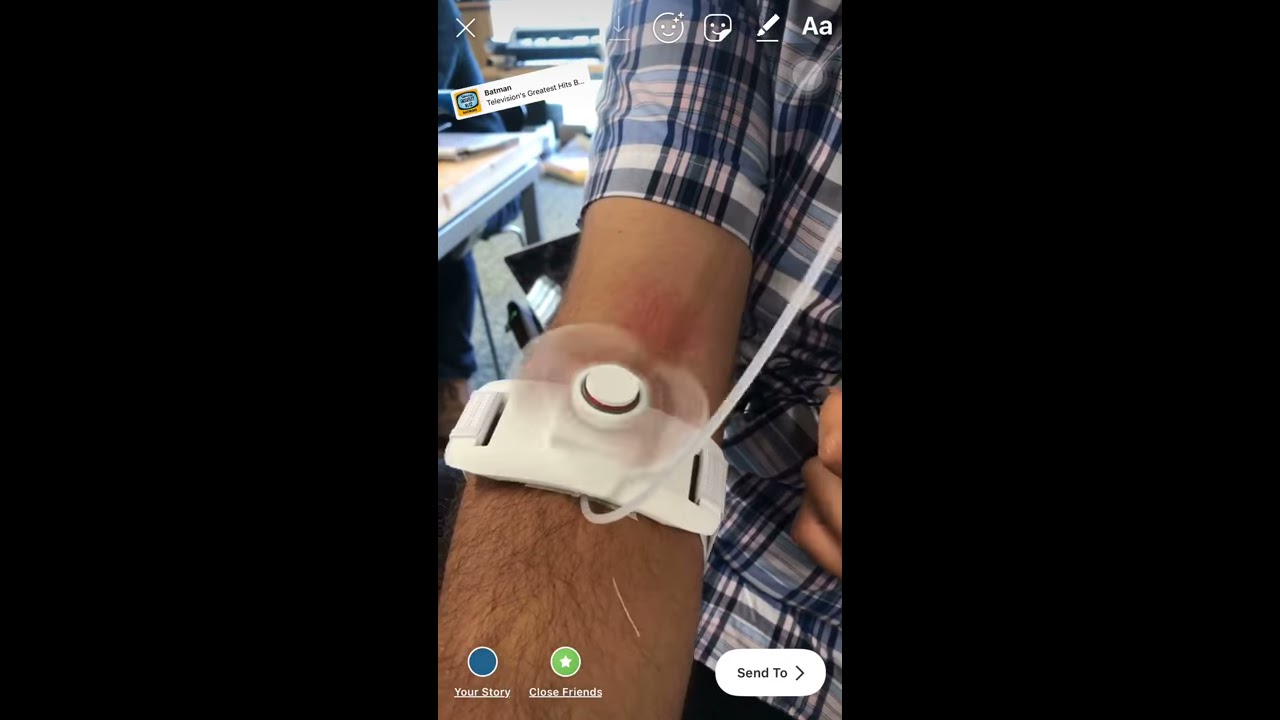This detailed image is a close-up photograph in portrait orientation of a man's right arm, prominently outstretched and centered against a black landscape background. He is wearing a blue and white checkered short-sleeved shirt. Attached to the inner elbow of his arm is a white medical device, resembling a blood pressure monitor, with a wire extending upwards. Below the image, in the app interface, there are three navigational buttons. The left button is blue and labeled "Your Story." Next to it, the middle button is green with a white star in the center, labeled "Close Friends." On the far right, a white button displays "Send To" with a right-pointing arrow. The photo suggests an educational or clinical setting, emphasizing the details of the medical device and app interface elements.